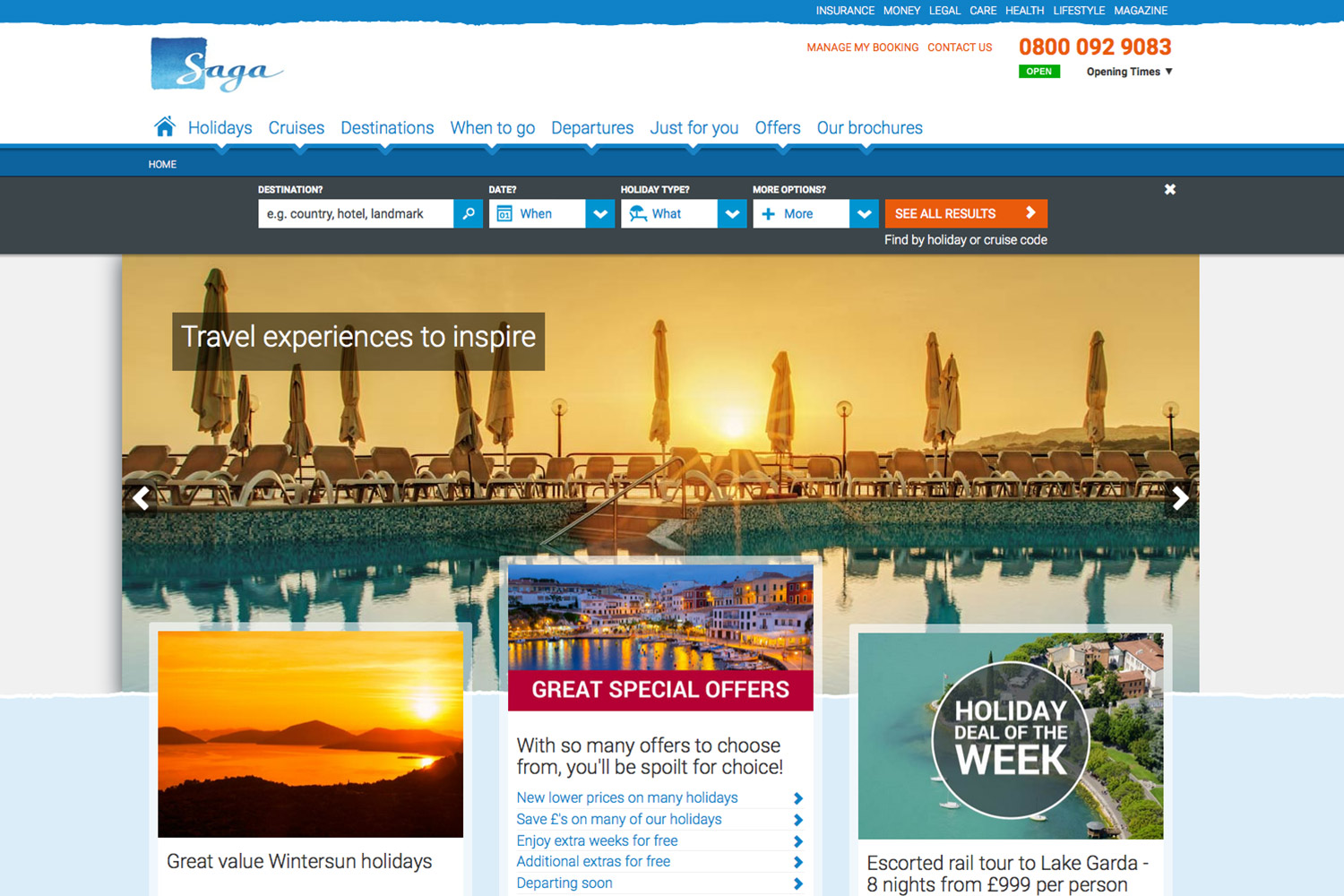The image depicts a travel website branded "Saga" prominently displayed at the top left corner. The navigation bar features several tabs starting with a home icon, followed by options labeled "Holidays," "Cruises," "Destinations," “When to Go,” “Departures,” “Just for You,” "Offers," and "Our Brochures."

Below the navigation bar, there are multiple search fields designed for user input, with sections to enter details such as destination, date, holiday type, and additional options. At the far end of these fields, there's a prominent orange button labeled "See All Results."

Further down the page, there's a section that allows searches by holiday or cruise code. This emphasizes that the website specializes in cruises. Above these elements, a banner reads, "Travel Experiences to Inspire," suggesting a focus on enriching travel experiences. The image also shows a visual, perhaps of a luxurious pool, enhancing the appealing aesthetics of the site.